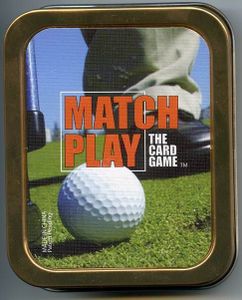This is an advertisement for "Match Play the Card Game" depicted within a brass rectangular frame with rounded corners. The main image features a golfer's left leg, dressed in khaki pants and a black shoe, standing on a putting green. Prominently displayed at the center is a white golf ball. The text "Match Play" is boldly written in all-capital red letters, while "the card game" is in smaller white type beneath it. The photograph also showcases part of a golf club with a blue shaft on the left side. The golden or amber-toned frame, possibly due to lighting effects, adds a vintage touch, suggesting the game's nostalgic appeal, likely from the 90s.